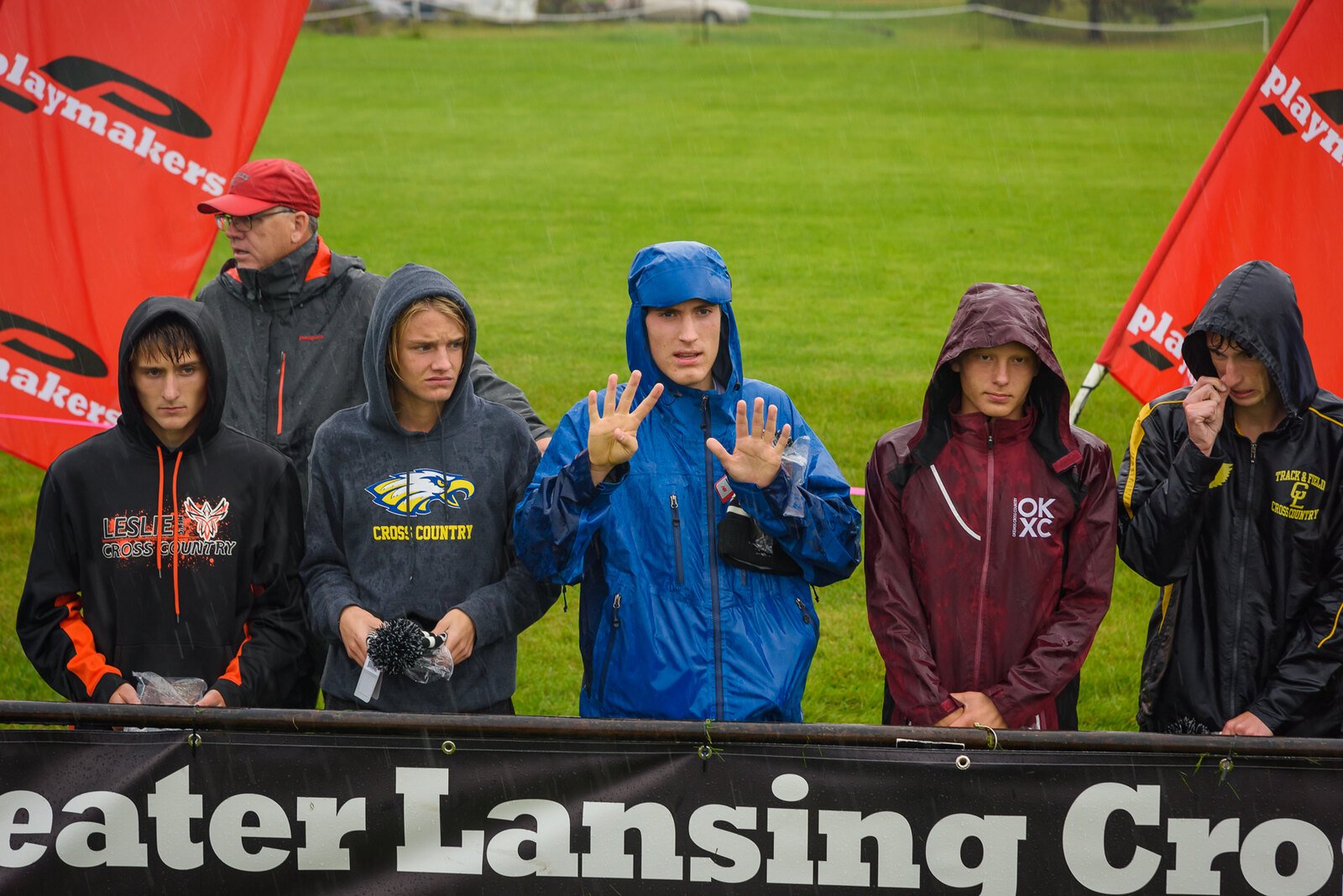This is a horizontally aligned rectangular picture capturing a group of six people, likely involved in a cross-country running event, standing behind a large black banner in the rain. The banner has partially visible text in white, which appears to spell out "Lansing Cross Country." The event is taking place on a lush, green grassy field. 

To the left and right upper corners of the image, portions of red flags can be seen, each displaying a large black "P" and the word "Playmakers" in white. 

The individuals in the photograph include five young people and one adult standing behind them, possibly a coach. The central figure among the youths is holding up nine fingers and wearing a blue hooded jacket. To his left is a young lady in a yellow hoodie featuring an eagle and the words "Cross Country." Next to her is another student in a black and orange hoodie with "Leslie Cross Country" written on it. The person furthest to the left is a young man in a gray hoodie.

On the right side of the central figure, there are two more young men. One is in a burgundy zippered hoodie with "OKXC" in white letters; the other is wearing a black and yellow hooded jacket with "Track and Field Cross Country" on it and appears to be scratching his nose.

Behind these youths stands an adult male, presumably a coach. He is wearing glasses, a red ball cap, and a gray and orange jacket, looking towards the left. Despite the rain, evident from their damp appearances and raised hoods, the group appears engaged and ready, hinting at their dedication and enthusiasm for the event.